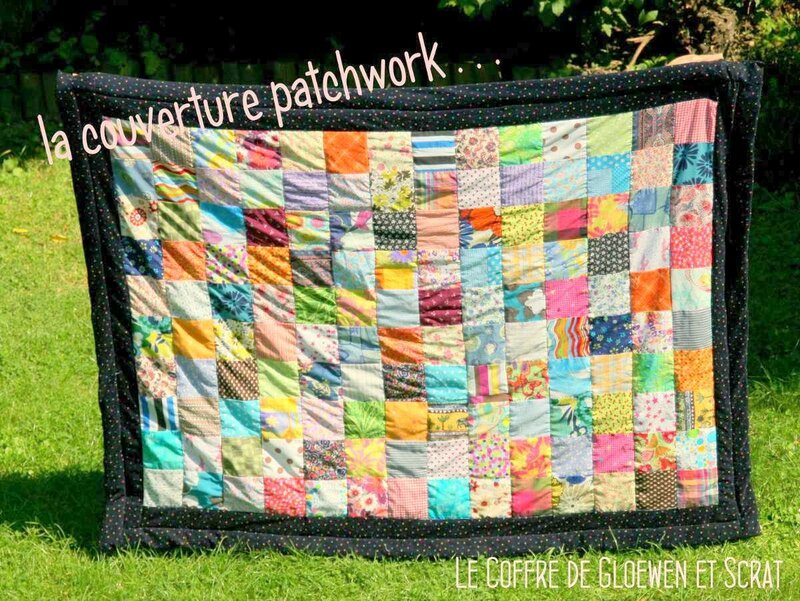The image depicts a vibrantly colorful quilt displayed against a background of lush green grass and dense foliage, suggesting it might be in a backyard or park. The quilt is held up by an unseen frame or a clothesline, creating a flat, expansive view. The quilt itself features a prominent black border adorned with polka dots. Inside, there are 10 vertical by 14 horizontal rows of fabric squares, each showcasing a variety of colors and patterns, ranging from pastel hues to bold designs that include dots, flowers, and geometric shapes. At the top left corner of the quilt, the text "LA COUVERTURE PATCHWORK..." is printed in white or pink, while in the lower right corner, "LE COFFRE DE GLOEWEN ET SCRAT" is also displayed in matching text. The image highlights the intricate artistry and detailed patterns of the quilt amidst a serene natural setting.